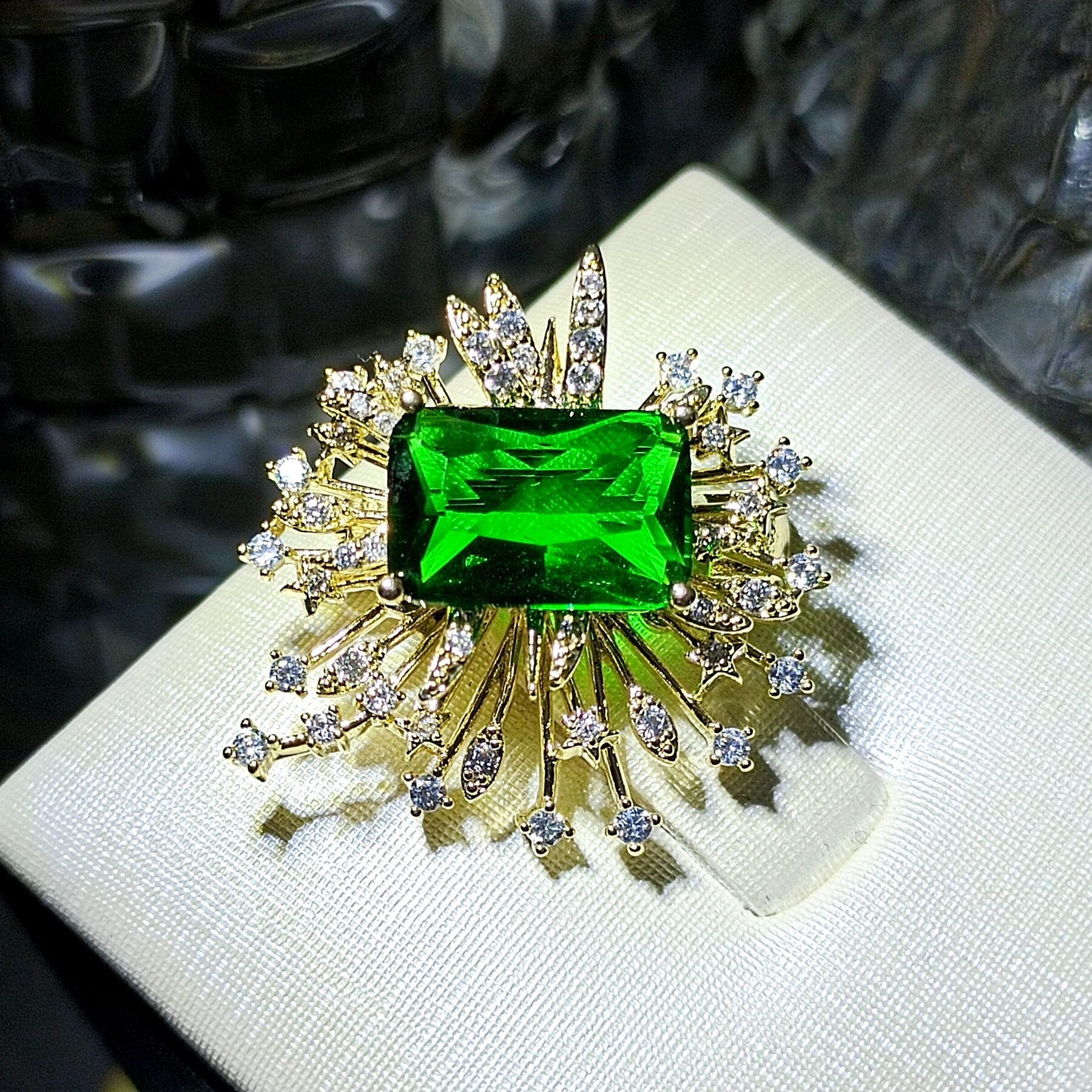The image depicts an intricately designed piece of jewelry set against a black background, adorned with white swooshes that lend an out-of-focus, almost ethereal quality to the backdrop. Central to the composition is a radiant gem of emerald green, encased in a sunburst pattern of lines that emanate outward. These lines appear to be crafted from a combination of gold and silver, culminating in a dazzling array of diamond-like shapes at their ends. The jewelry rests on a form-fitting insert, possibly of a jewelry case, covered in a white, cross-stitched material. A small bump in the middle of the insert creates a subtle protrusion, adding depth to the display. This elegant arrangement highlights the jewel’s brilliance, making it the focal point of the image.